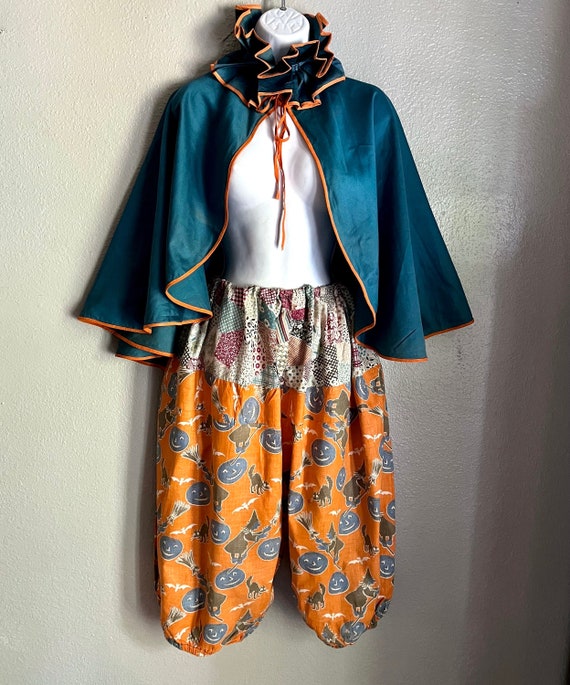The photograph features a mannequin attached to a white-washed wall, with some shadows visible on the right side, possibly cast by the outfit itself. The mannequin, primarily showing only the torso up to the neck, appears to be female. The outfit includes a striking green cape draped around the neck, adorned with green borders. The mannequin's body is dressed in a white top paired with loose, comfy-looking pants that have an orange base color. The pants are decorated with playful patterns that include a sun, a cup, and a rat. The scene is set against a plain white background, with a string attached to the neckline of the outfit, adding a final touch to the display.